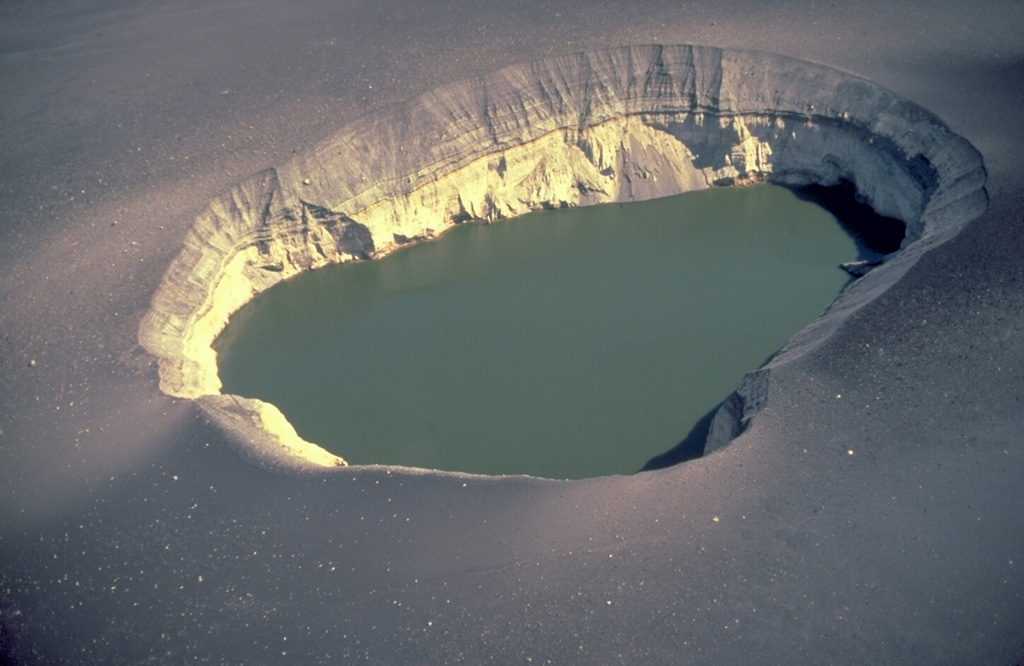The image depicts a large, oval-shaped pit with steep walls descending to a body of murky, dark green water at its base. The surrounding landscape is predominantly gray, with patches of soot-covered snow or grayish sediment, likely indicating a desolate or desert-like environment. The pit itself showcases distinct geological layers: the upper half is dark gray, transitioning to a lighter gray and whitish hue as it nears the water. This suggests sedimentary formations built over time. The water within the pit is perfectly still, adding to the eerie stillness of the scene. The contrast between the dark, cavernous pit and its lighter surroundings highlights the stark and surreal nature of this odd geological feature.